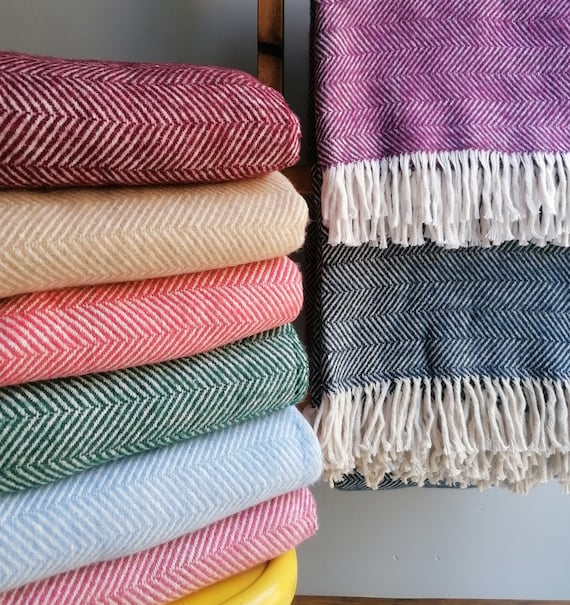This detailed photograph resembles an image from a catalog, potentially an IKEA or a towel manufacturer's website, showcasing a variety of woven beach towels and blankets. On the left-hand side, there is a neatly stacked pile of these towels placed on a yellowish table. The towels are arranged in the following order from top to bottom: maroon and white, peach and white, green and white, light blue and white, pink and white, and finally, a bottom towel in a pink and white combination.

To the right of this stack, two towels are hanging and exhibit distinct designs with white tassels. The top hanging towel is a purple and white blend, while the bottom hanging towel features a navy blue and white pattern. All towels share a unique design of arrows pointing upward, creating a textured and visually appealing pattern against a background that seems to be either concrete or light slate blue. The entire composition portrays an organized and colorful display, emphasizing the woven texture and intricate designs of the towels.